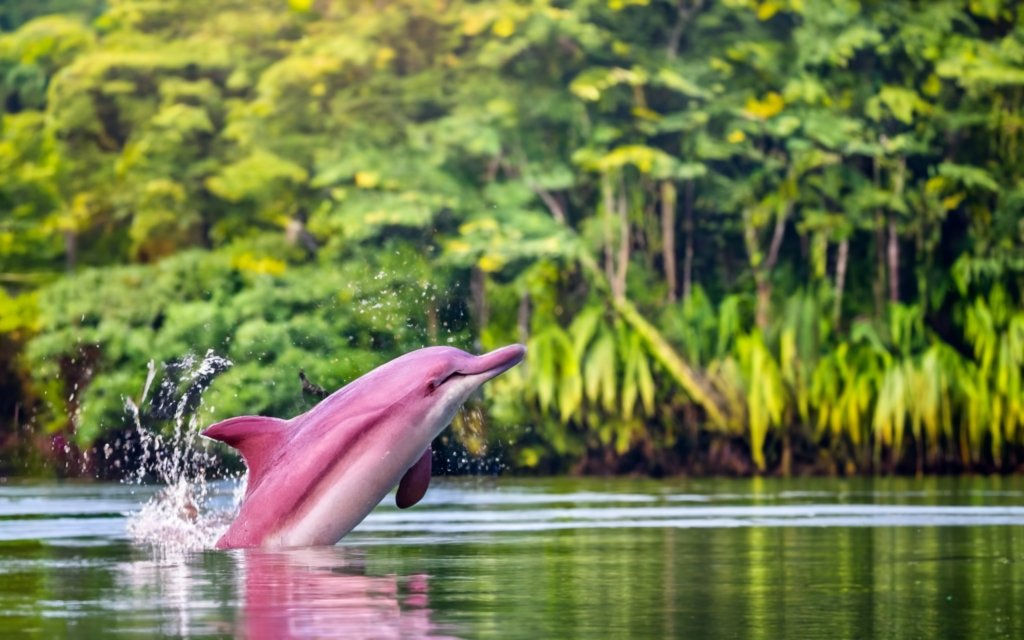The image depicts a striking, possibly AI-generated or heavily edited scene of a pinkish-red dolphin leaping out of a tranquil river, surrounded by dense, jungle-like foliage. The dolphin, with its unusual reddish-pink hue transitioning to a white underside, appears to be missing a fin on one side, and its mouth unnaturally extends too far back, cutting through its eye. Emerging about 65% from the water, the dolphin's tail fin remains submerged, creating splashes that trail behind and above it. The background is dominated by tall, thin trees growing right up to the water's edge, with no visible land, enhancing the impression of a river in an exotic, lush environment.